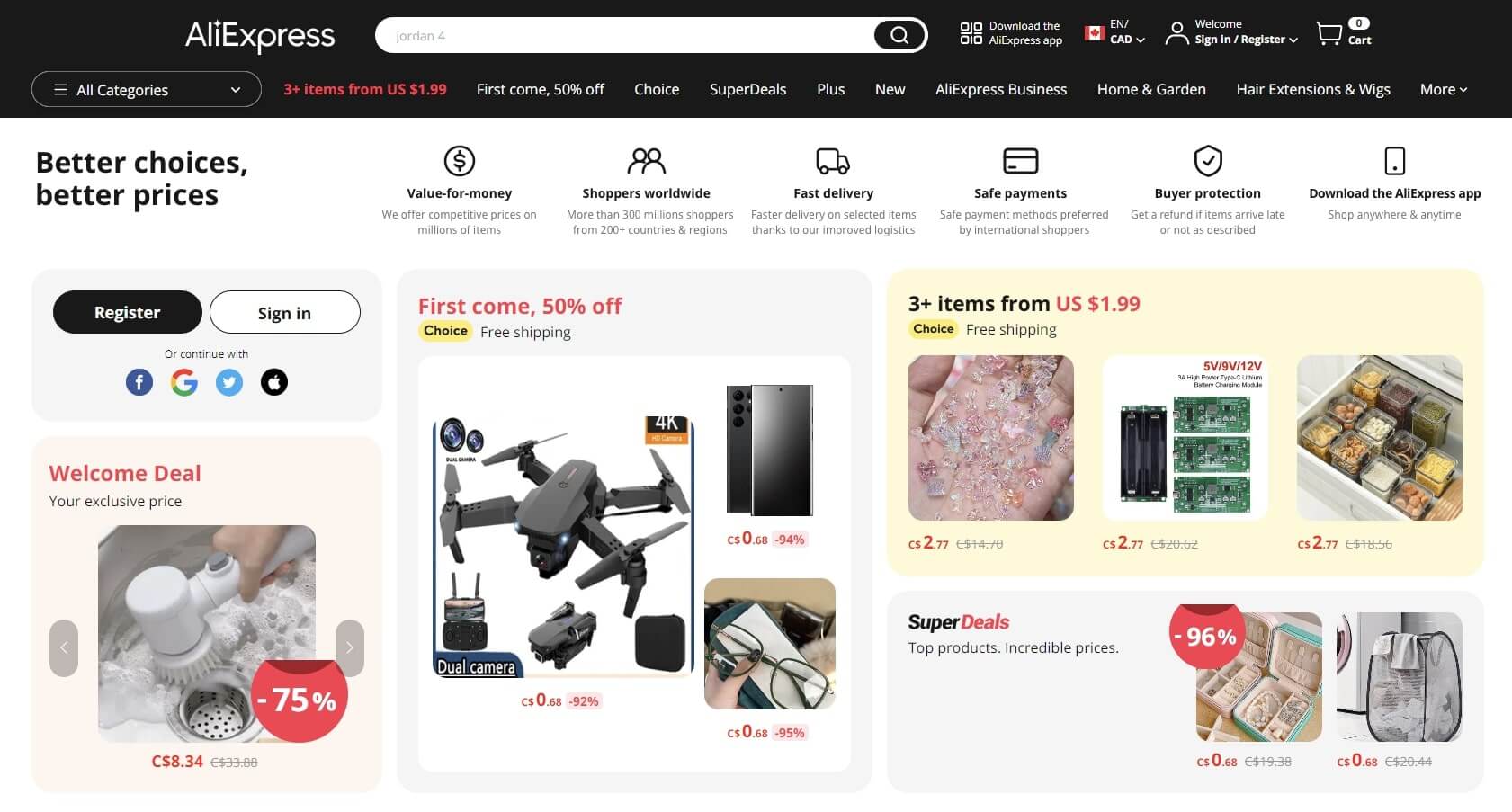In the image, there is a white background with a black header at the top displaying the AliExpress logo. To the right of the logo is a large white search bar. Adjacent to the search bar are icons including a red and white box, a shopping cart, an "All Categories" drop-down menu, and several navigation headings. Below the header, the white background features various promotional texts such as "Better choices, better prices," "Value for money," "Shoppers' variables," "Fast delivery," "Safe payments," "Buyer protection," and a prompt to download the AliExpress app.

Further down, there is a blue box containing a black "Register" button and a white "Sign In" button, accompanied by icons for social media platforms like Facebook, Google, and Twitter. Below this, a pink box with the text "Welcome Deal: Your Exclusive Price" advertises a 75% discount. In the center of the image, a larger blue box promotes a "First Come, First Serve" deal with a 50% discount and free shipping on three highlighted items. On the right side, another pink box showcases a deal for purchasing three or more items starting from US $1.99, displaying images of three different products. Lastly, the image highlights "Super Deals" with up to 96% off on two specific items.